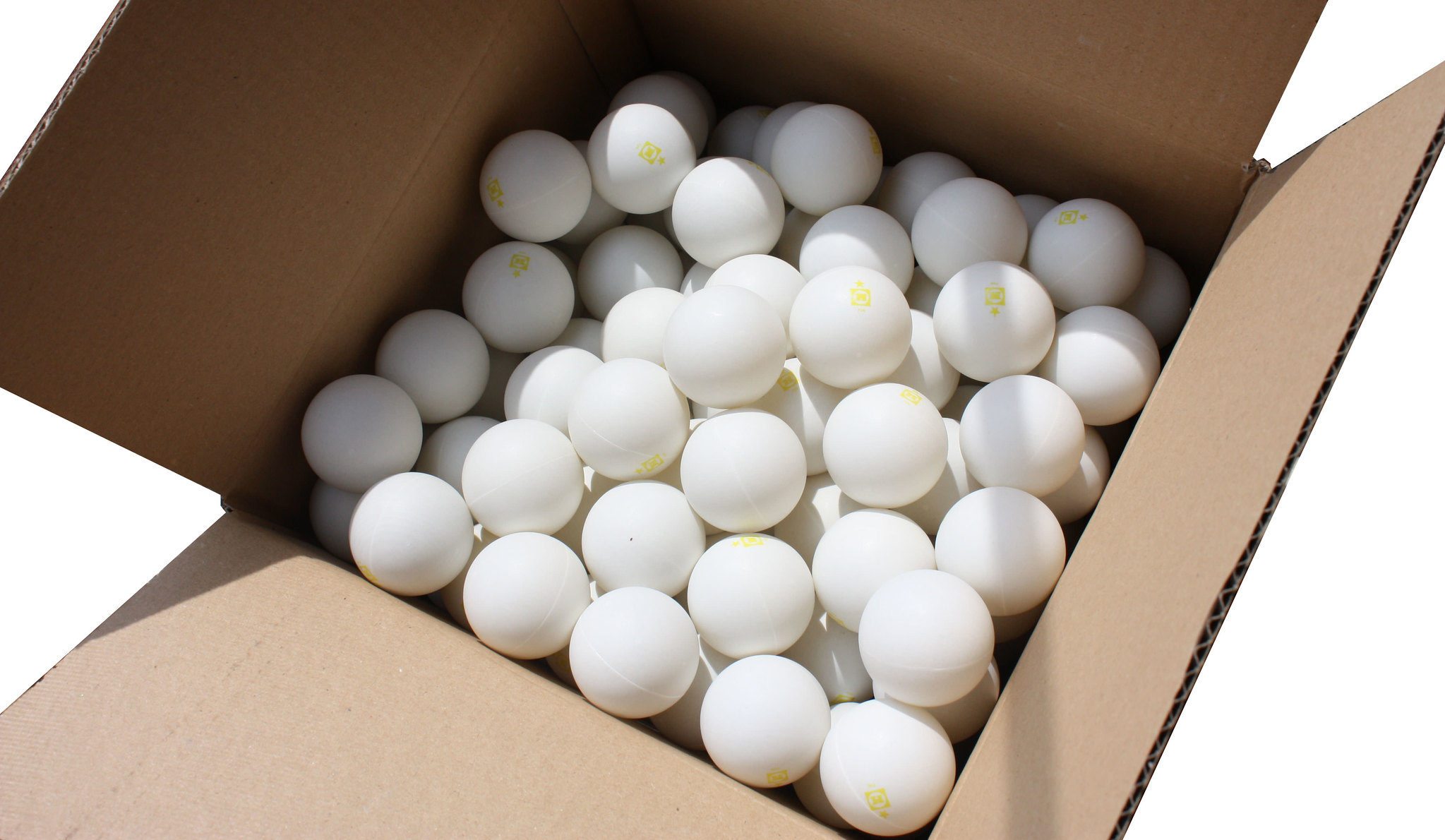The photograph captures a cardboard box filled to the brim with what appears to be dozens of small, white ping-pong balls. Shot from above, the image shows the box flaps upright against a blank white background, emphasizing the simplicity of the scene. The box is sturdy and rectangular, roughly measuring 12 by 12 inches in width and 8 inches deep. The ping-pong balls within the box are almost uniform white, with some displaying faint yellow markings, likely logos or stamps. These yellow marks are subtle and not easily identifiable. The balls exhibit a slight seam, suggesting a plastic material. Shadows cast upon two of the box flaps create a subtle contrast against the lit ones, adding a hint of depth to the straightforward composition.